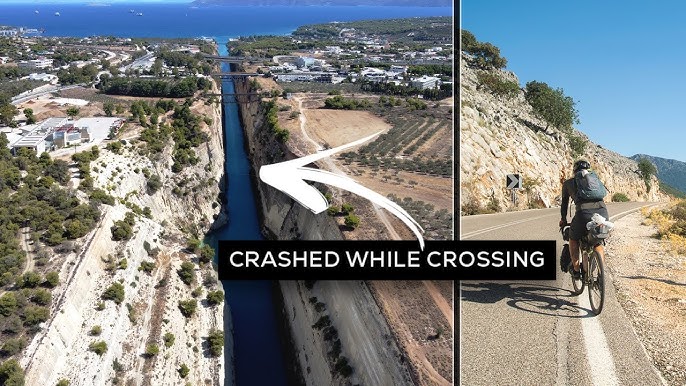This horizontally aligned rectangular image consists of two juxtaposed photographs. The left picture, a square aerial view, displays a narrow body of water running vertically from the bottom to the top, opening into a larger body of water at the top. Land flanks both sides of this waterway, featuring rocky terrain and clusters of trees, with some buildings visible near the top. A prominent, hand-drawn white arrow points to a specific spot in the middle of the water. Overlaying both pictures is the bold, all-caps white text "CRASHED WHILE CROSSING" set against a black rectangular background. 

The smaller, right-hand image provides a close-up view of a cyclist seen from behind, riding a 10-speed bicycle along a road adjacent to a mountain. The cyclist is equipped with a helmet, backpack, and water bottle, while other essentials are stored in the bike's rear basket. The overall scene, captured in vivid colors such as light blue, dark blue, gray, tan, off-white, black, light green, and dark green, appears to be taken outdoors during the daytime.